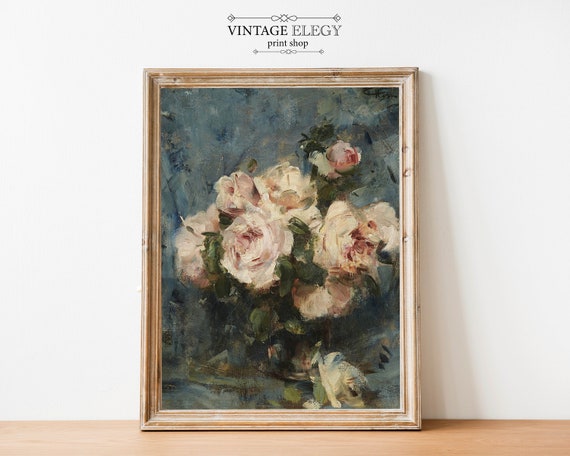In the image, there's a detailed framed painting showcasing a bouquet of pinkish-white roses set against a blue background. The painting adopts an impressionist style, characterized by thick brush strokes that leave the roses and leaves without much intricate detail. The bouquet features around six roses, some of which are in bud form, notably one in the upper right part of the painting. This framed canvas, encased in a light brown wooden frame, is leaning against a white wall rather than being hung. Above it, the words "Vintage Elegy Print Shop" are clearly visible. Additionally, the painting rests on a light brown, wood-grained surface at the bottom.